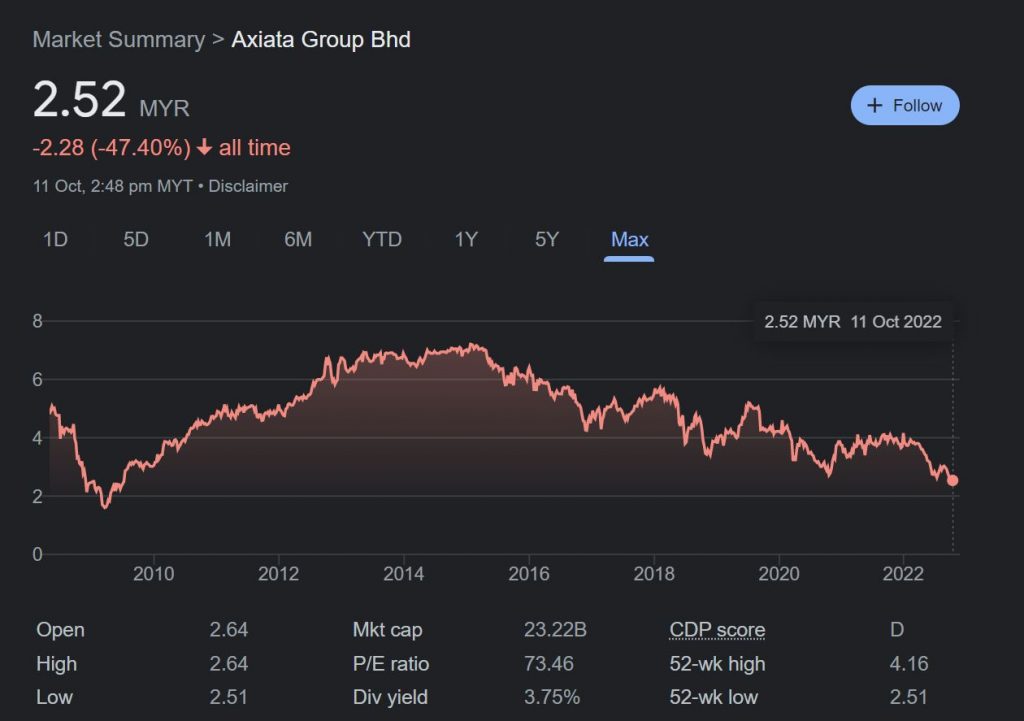This is a detailed screenshot of a stock price graph for Axiata Group BHT, presented with a black background. At the top right corner, there is a blue "Follow" button. The graph is titled "Market Summary: Axiata Group BHT" and indicates that the current stock price is $2.52 MYR, reflecting a significant decrease of 2.28 MYR or approximately 47% from its all-time high.

The data is timestamped at 2:48 p.m. MYT on October 11th. The chart displays the maximum price data over time, with the x-axis ranging from the year 2010 to 2022 and the y-axis spanning from 0 to 8 MYR. Key financial metrics provided include an opening price of $2.64 MYR, with the day's high also at $2.64 MYR and a low of $2.51 MYR.

Furthermore, the market capitalization is noted at $23.22 billion, with a Price-to-Earnings (P/E) ratio of 76.46. The dividend yield is listed at 3.75%, and the CDP score stands at a D. Over the past 52 weeks, the stock reached a high of $4.16 MYR and a low of $2.51 MYR.